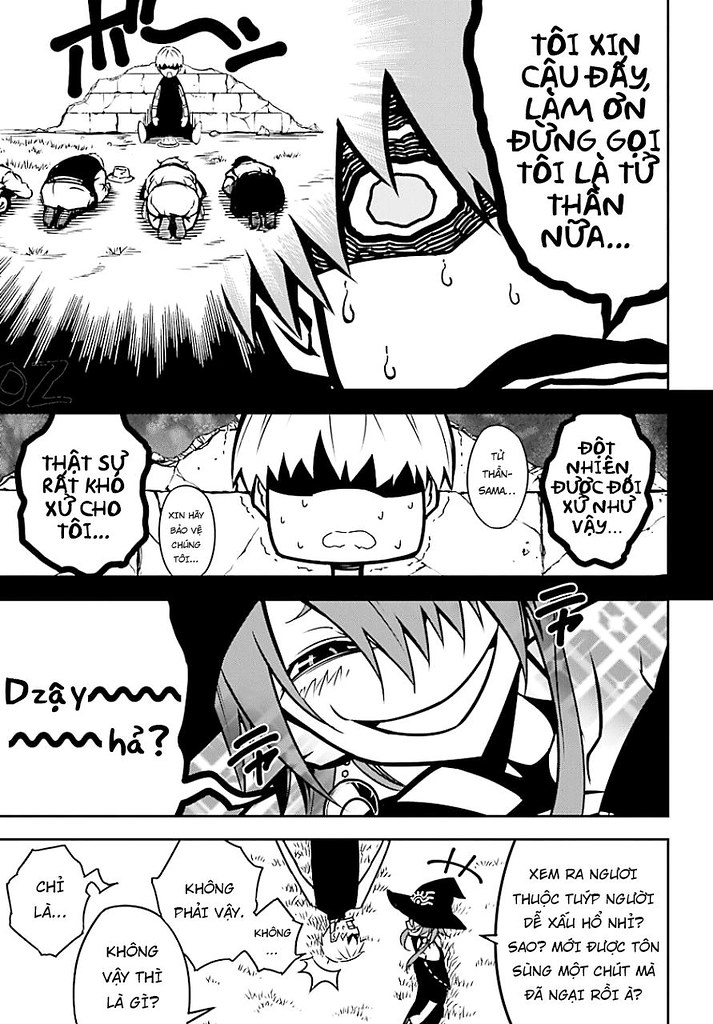The image depicts a black-and-white manga page split into four panels, each filled with text bubbles in an unfamiliar language. In the top panel, a character sits cross-legged in front of a broken brick wall with a mountain visible in the background. Three other characters are bowing deeply before this seated figure, who appears shocked and confused by their actions. The second panel shows a flustered character with bangs covering their eyes and sweat drops around their face, accompanied by multiple text bubbles. The third panel features a grinning character facing the viewer, their smile wide and mischievous, with hair covering one eye. The bottom panel portrays a whimsical scenario with someone hanging upside down, engaged in conversation with a person wearing a witch's hat. Both characters are surrounded by further dialogue bubbles, hinting at a comedic and quirky narrative unfolding.